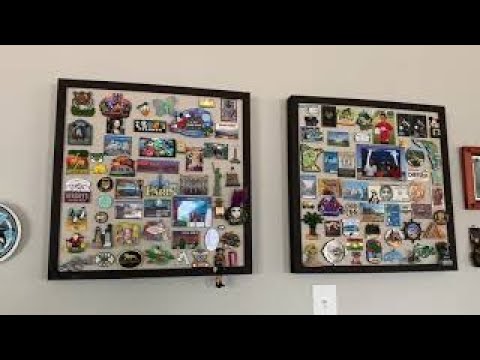The photograph features a bright, off-white or light gray wall adorned with various picture frames. Prominently displayed are two large, black-framed images, each containing around 50 to 60 colorful patches; these patches may be souvenirs, keychains, or badges, showcasing a blend of yellows, blues, and reds, though their exact details are somewhat blurred due to the distance and zoom level. Below the right frame, there is a white light switch. Adjacent to both large frames, partially visible on the sides of the photo, are more frames—one with a wooden border above and another with a black border below. Near the left black-framed patches, a circular object resembling a bowl is slightly visible, also mounted on the wall. The overall image is well-lit with natural light, contributing to a clear, colorful depiction despite some blurriness in the finer details.